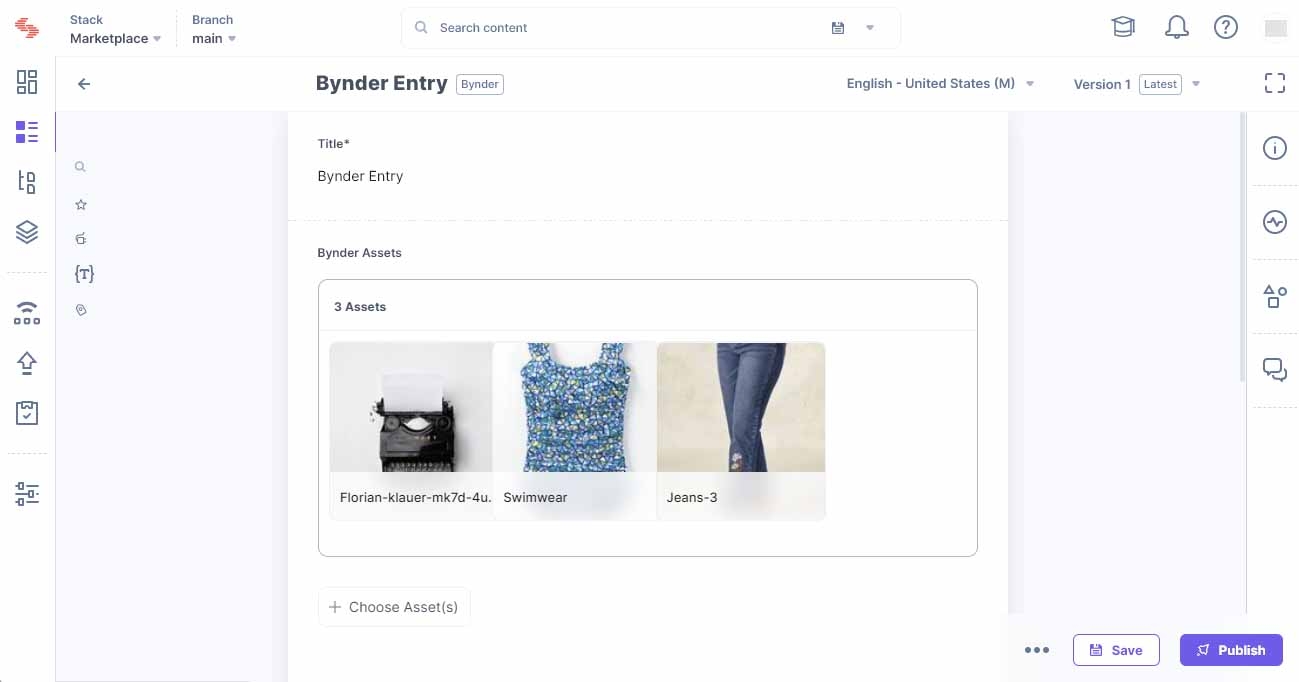The image displays a website interface with various elements and icons. In the top left corner, there's a red logo accompanied by two arrows—one pointing to the right, the other to the left. To the right of the logo, there are two tabs labeled "Stack Marketplace" and "Branch Main," respectively. 

Centrally located at the top is a search bar with a magnifying glass icon on its left. The placeholder text inside the search bar reads "Search Content," and to the right of the search bar is a floppy disk icon, followed by a gray downwards-pointing arrow.

In the middle of the page, the word "Binder" is prominently displayed, spelled "B-Y-N-D-E-R." The term "Binder Entry" is written next to it. Below this heading, it reads "Title * Binder Entry," followed by "Binder Assets" and the phrase "Three Assets." Underneath this section, there are images representing three different items.